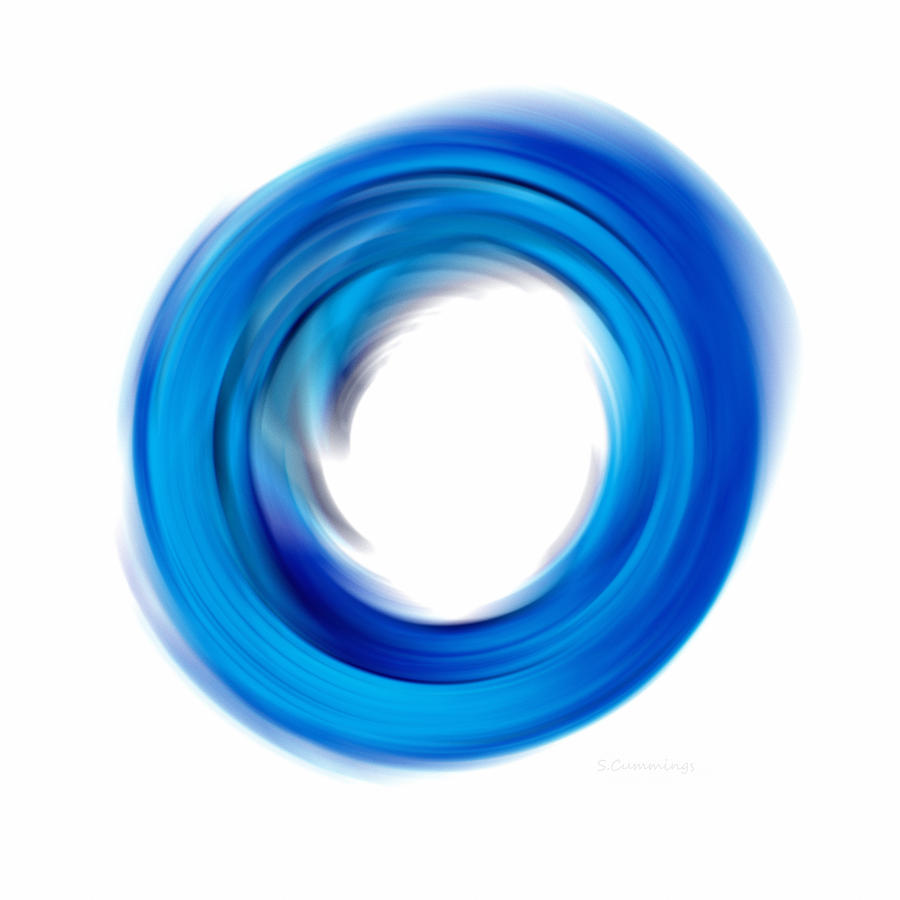The image features a blue, swirling circle on a white background, capturing a sense of rapid motion. The circle itself is composed of varying shades of blue, from dark blue to lighter blue with hints of gray, creating a dynamic blend that resembles paint being mixed together with a brush. The outer and inner borders of the circle are blurred, enhancing the impression of high-speed rotation. The circle's center is pure white, possibly reflecting light. There are darker portions on the outer edges that gradually transition to lighter shades towards the center, adding depth and movement to the swirl. The overall effect is a blur of colors and motion, creating an abstract, indistinct form that suggests both the chaotic patterns of a brushstroke and the centrifugal force of a rapidly spinning object.